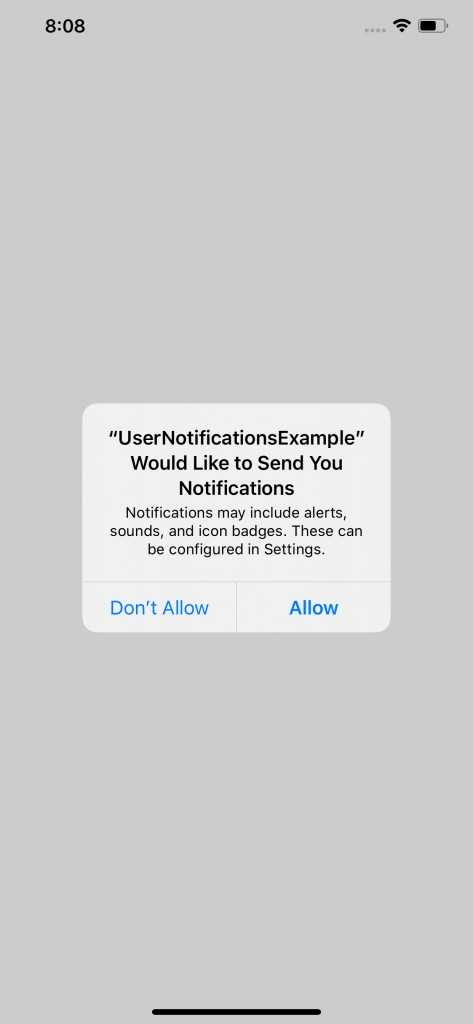Screenshot Description: 

The image is a screenshot taken from a cell phone displaying a notification prompt. At the top of the screenshot, the status bar indicates the time is 8:08 (without specifying a.m. or p.m.), along with icons for Wi-Fi signal strength and battery status, located at the top right corner.

The majority of the background is a uniform gray, providing a neutral backdrop for the central element of the image: a prominent white box with bold black text. This dialog box reads, "User Notification Example," enclosed in quotation marks.

Below this heading, the message continues, "would like to send you notifications. Notifications may include alerts, sounds, or icon badges. These can be configured in settings." 

At the bottom of the white box are two options for the user to select from: "Don't Allow" and "Allow," written in blue text.

The rest of the screen remains uncluttered, with a single, thin black line visible at the bottom center, possibly part of the navigation interface of the phone.